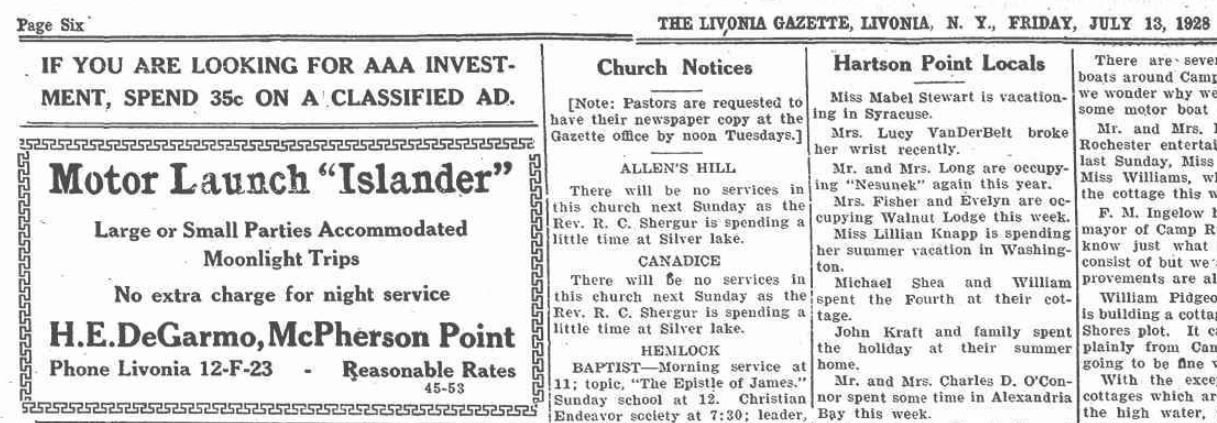This image features a scan of page six of the Livonia Gazette newspaper, dated Friday, July 13, 1928, from Livonia, New York. The paper is white with black print. On the left side, there's a prominent advertisement reading, "If you're looking for a AAA investment, spend 35¢ on a classified ad." Below this ad, another advertisement for "Motor Launch Islander" offers services for large or small parties, boasting moonlight trips at no extra charge for night service, managed by H.E. DeGarmo from McPherson Point with reasonable rates.

To the right of these ads, a column labeled "Church Notices" includes a note requesting pastors to submit their newspaper copy by noon on Tuesdays. It mentions that there will be no services at Allen's Hill church next Sunday as Reverend R.C. Sugar will be spending time at Silver Lake. Additionally, the Hemlock Baptist church will have a morning service at 11 a.m. with the topic "The Apostle of James," followed by Sunday School at noon and a Christian Endeavor Society meeting at 7:30 p.m.

Further to the right, an article titled "Hartson Point Locals" lists various personal updates: Miss Mabel Stewart is vacationing in Syracuse; Miss Lucy Vanderbilt recently broke her wrist; Mr. and Mrs. Long are back at Nesnook; Miss Fisher and Evelyn are staying at Wallout Lodge for the week; Miss Lillian Knapp is spending her summer vacation in Washington; Michael Shea and William commemorated the Fourth at their cottage; John Kraft and his family enjoyed the holiday at their summer home; and Mr. and Mrs. Charles DeConner visited Alexandria Bay this week. The article continues with more local updates, though part of the column is cut off.